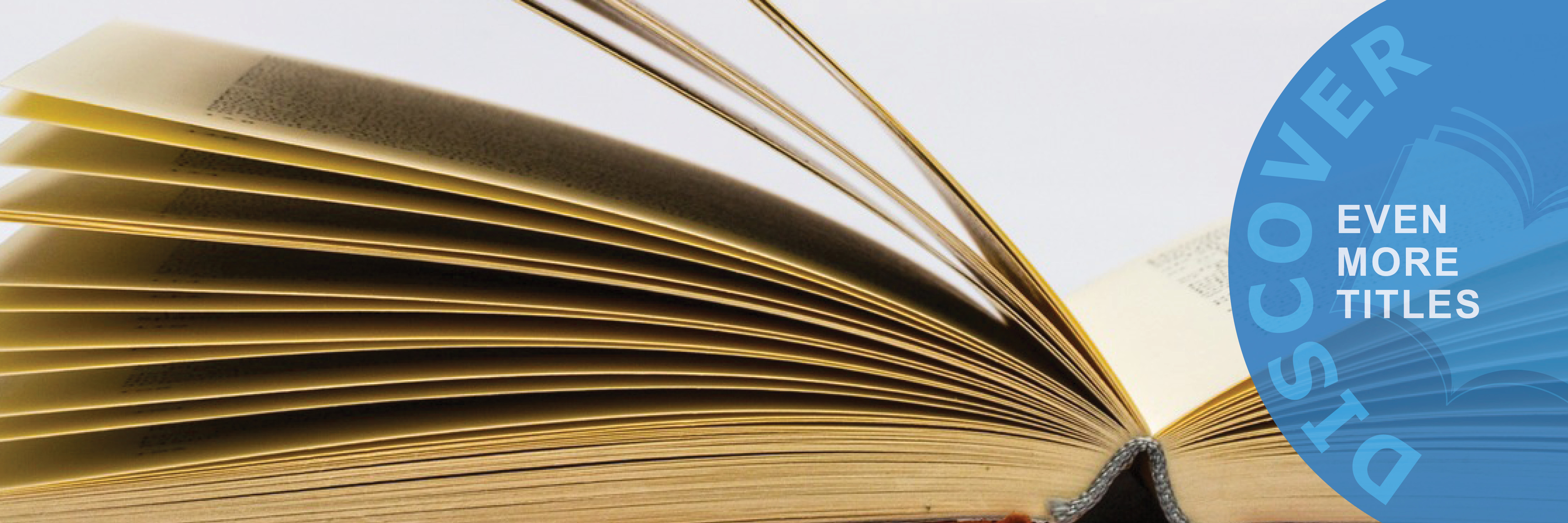The image depicts a landscape layout photograph of an old, hard-covered book that is halfway open and positioned against a stark white background. The book's gray cover has white speckles, and its pages, which appear weathered white and slightly raised, reveal glimpses of black text. The left side of the image shows the bottom pages closely packed together, while the upper pages fan out more due to the book's crease. To the right of the book, there is a prominent blue semi-circle featuring the word "Discover" in light blue text, and beneath it, "even more titles" in white text. The semi-circle creates a transparent effect, allowing the viewer to see the open pages of the book through it. The photograph appears brightly lit, with strong light bathing the book and the background, creating a highly illuminated scene.